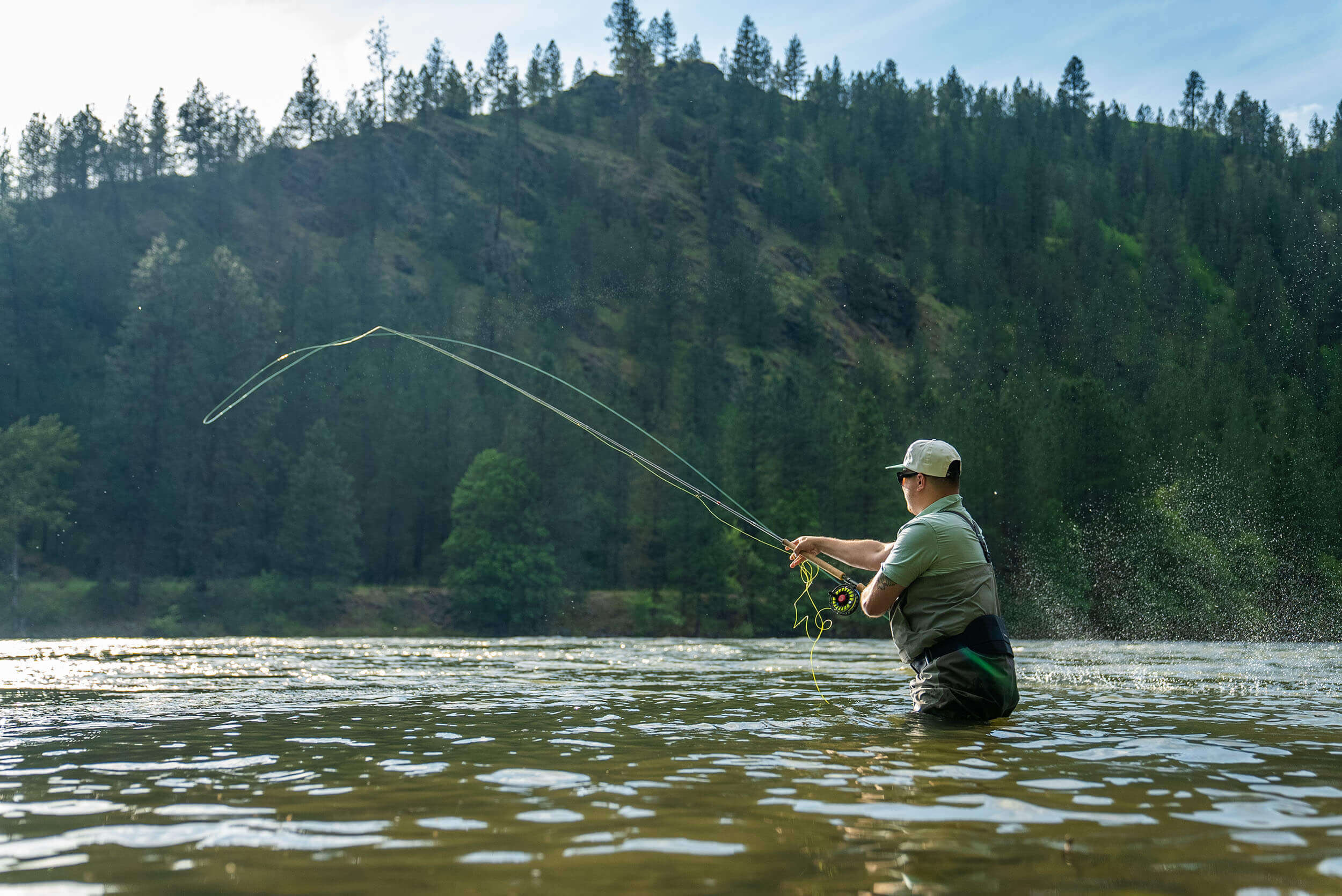In this detailed outdoor photograph taken during the daytime, a man is captured mid-action while fly fishing in a body of water, which could possibly be a river or lake. The rectangular photograph measures approximately six inches in width and four inches in height. The water, occupying the lower portion of the image, is a light brownish-green color with hints of blue in the wave peaks due to the sunlight. The man, positioned on the right side and standing about thigh-deep in the water, is of Caucasian descent and has a heavier build. He is donning a light gray baseball cap, dark sunglasses, a light green short-sleeved shirt, and gray pants or waders along with a black waistband or possible back brace. With a long fishing pole extended in front of him, he appears to be engaged in fly fishing, evidenced by the long, whipping line. Behind him, dispersed water droplets suggest recent, vigorous casting.

The backdrop features a tall mountain or hill, lush with dark green pine trees, and spans the entire width of the middle and upper sections of the image. The sky above shows a gradient, transitioning from deep blue on the right to nearly white on the left, possibly due to the brightness of the sun or clouds overhead. This scene beautifully captures the serene yet dynamic nature of fly fishing in a picturesque wilderness setting.